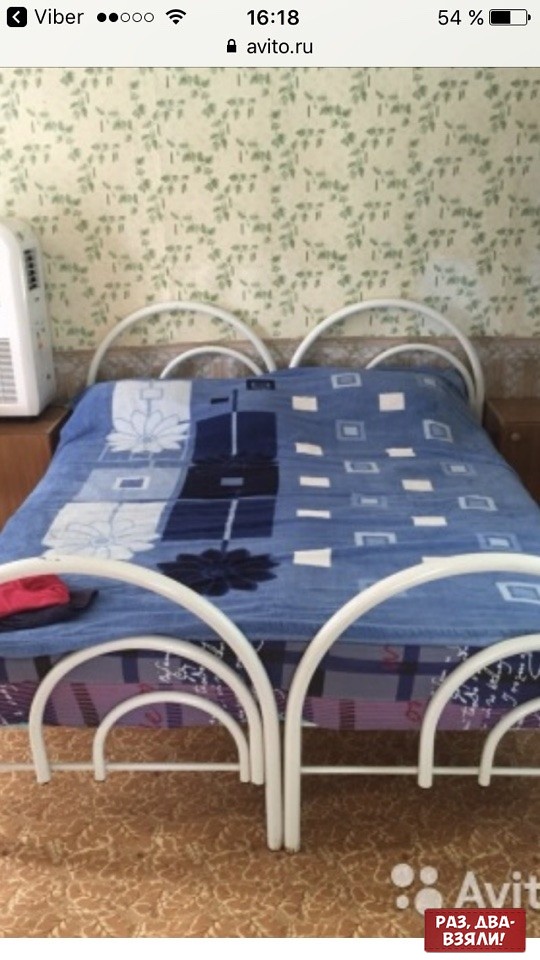This image appears to be a screenshot taken from a smartphone, possibly an older iPhone model. At the top, the interface displays elements indicating the device's status: the network carrier "avito.ru," the Wi-Fi connection labeled as "Viber," two signal bars, a battery level of 54%, and the time at 16:18. 

Central to the image is a full-size or queen bed with a distinctive white metal headboard and footboard, each forming a graceful swooping shape that resembles the letter "M." The bed is dressed with a blue bedspread that features a variety of patterns, including large squares on the left side with white and dark blue flowers, and smaller squares on the right. This mix of designs adds visual interest to the ensemble.

The background showcases a wallpaper adorned with off-yellow tones and green leafy patterns, complementing the natural theme extending onto the floor, which is decorated with a pattern resembling leaves in shades of light and medium brown, giving a textured appearance. In the corner of the image, a white object is partially visible, though its exact nature remains unclear.